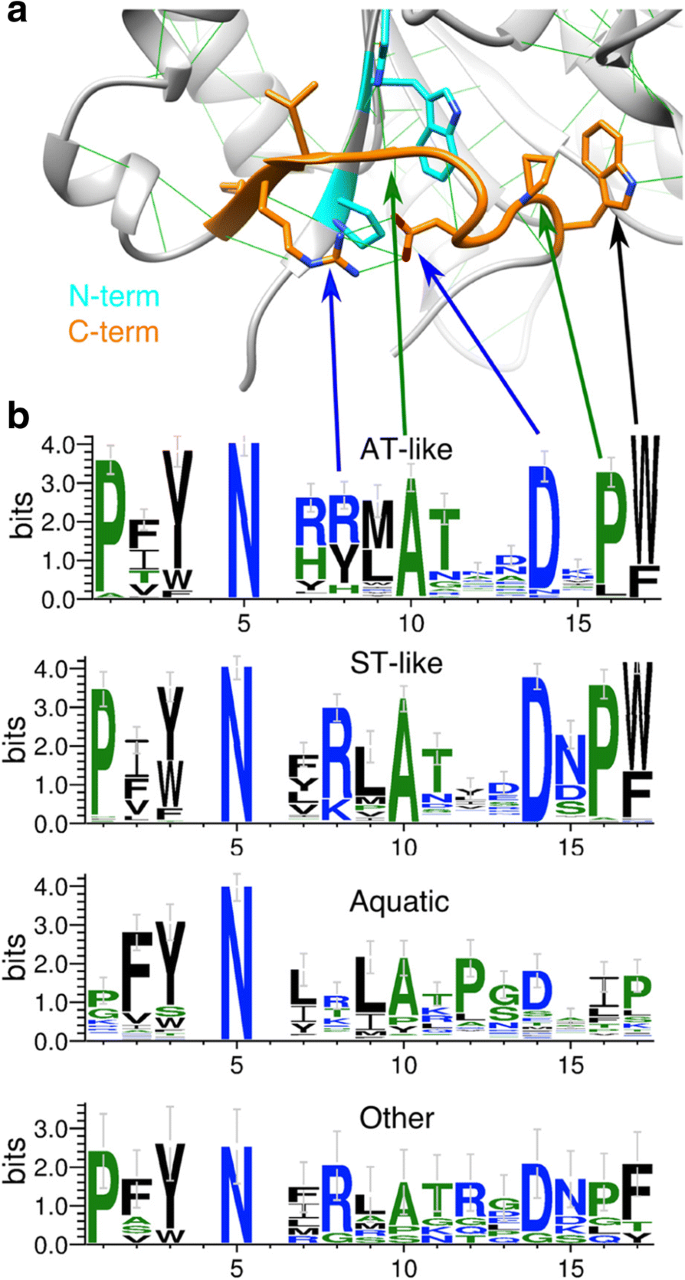The image is a detailed, colorful chart that resembles an old textbook illustration from possibly a century ago. It comprises four distinct charts labeled A and B, where each chart is marked with the term "bits" and numerical scales going from 0.0 to 3.0. The charts are also accompanied by a series of confusing and seemingly random letters such as P, F, Y, N, and C-term and N-term, which appear to be related to mathematical or scientific data, possibly genetic codes.

At the top of the chart, there are intricate, indescribable squiggles and art-like markings with arrows pointing toward them, which could suggest some form of complex model or corrupted file that didn’t print correctly. Diagram A features a complex model with squiggles, cylinders, triangles, and color-coded segments (orange, red, blue, cyan), and labeled as N-term and C-term. Diagram B includes various types of graphs such as AT-like, EST-like, and quarter graphs, each presenting structures with a column labeled "bits" on the left going up to 4.0. These diagrams are cluttered with obscure words and labels pointing towards different segments, contributing to an overall sense of complexity and confusion.